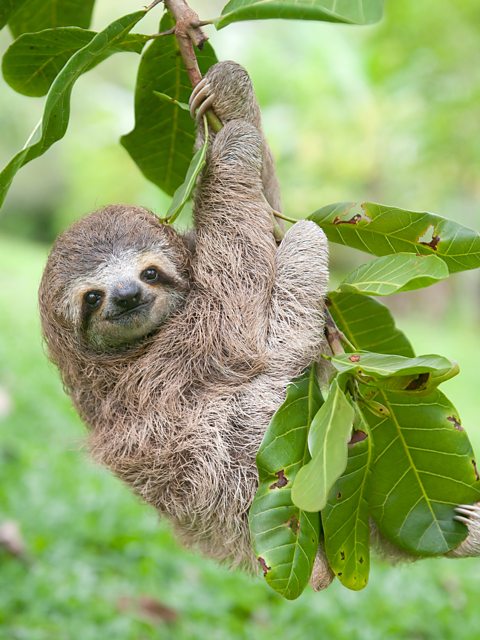This is a detailed close-up image of a sloth hanging from a branch of a tree. The sloth, with its long, sharp claws, grips the branch that is adorned with large, thick, green leaves, each leaf featuring a lighter green central vein with vascular bundles extending outward. The sloth, exhibiting a mix of grey, brown, and white fur, appears to have a small grin on its face and is staring directly at the camera. Its face is mostly white with distinctive black streaks extending from its black eyes down to the jawline. The background is beautifully blurred, showcasing a lush green environment with various trees and undergrowth that indicate a natural, forested habitat. The sloth's prominent nose and messy fur, which is darker around the head and lighter towards the bottom, add to the detailed serenity of the scene.